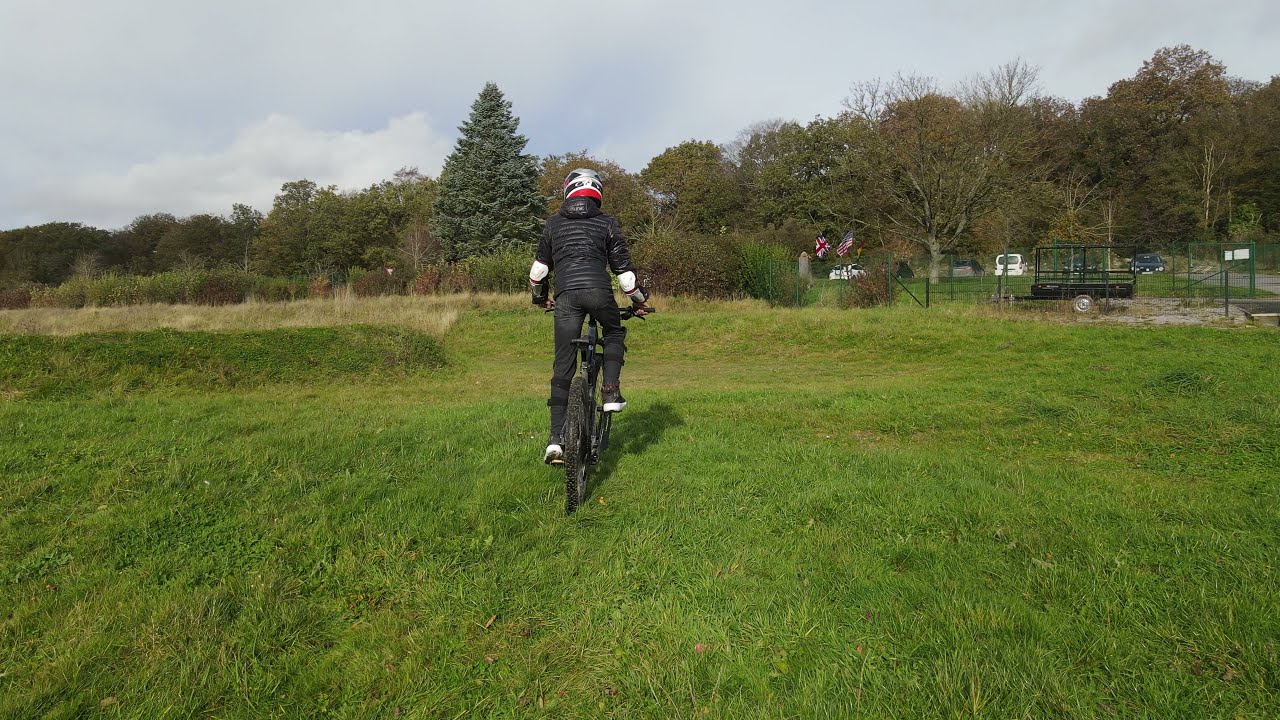The image depicts a lush, green, grassy field extending into the distance, featuring a solitary individual riding a bicycle away from the camera. The cyclist is dressed predominantly in black, wearing a black jacket, black pants, dark-colored shoes with white soles, and protective gear including a helmet that has white accents, elbow pads, and knee pads. The cyclist is riding on thick grass, seemingly attempting to ascend a gentle hill. To the right side of the scene, there appears to be a trailer, some wheels, fencing, a possible house, and various vehicles. The background is framed by a strip of trees, including pine trees and other varieties, that stretch from the left to the right side of the image. Above this serene outdoor setting, blue-gray skies dotted with fluffy white and gray clouds complete the picturesque landscape.